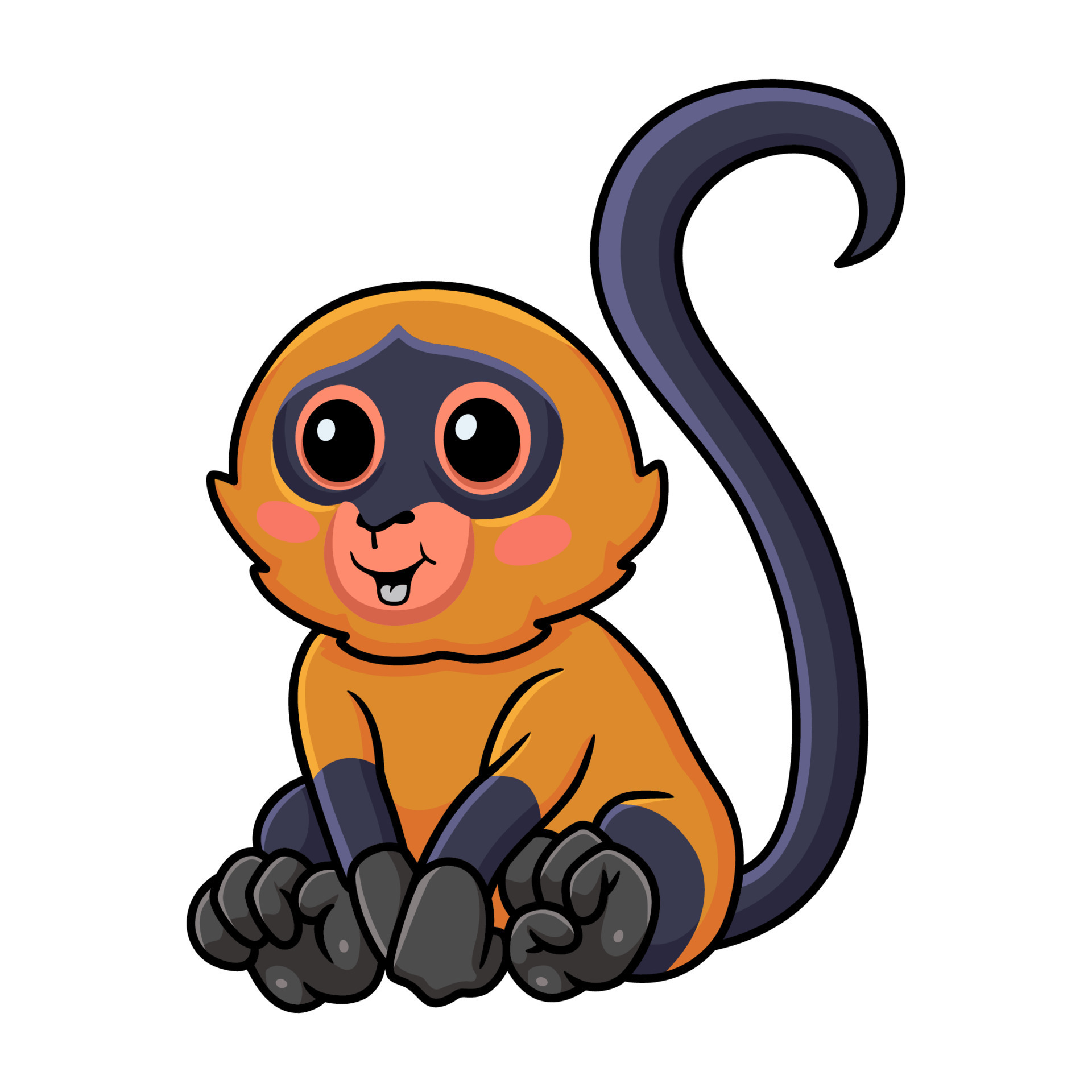In a low-resolution cartoon or clip art image, we see a small, young monkey depicted with a charming blend of colors and intricate details. The monkey's overall body is a vague orangish-brown hue with black hands and feet, accentuated by patches of dark blue above them. Its long, blue tail, which extends beyond the length of its body, adds a distinctive feature to its appearance. The monkey is seated with its feet in front and hands clasped together between them, creating an endearing pose. Its wide-open black eyes, dotted with white highlights to indicate light reflection, are surrounded by raccoon-like patches of dark blue, giving it a mischievous look. The pink circles on either side of its open mouth suggest blushing, enhancing the impression that the monkey is either smiling joyfully or feeling a bit embarrassed. The outline of the drawing is rendered in black, providing a clear and defined edge to this vividly expressive monkey.